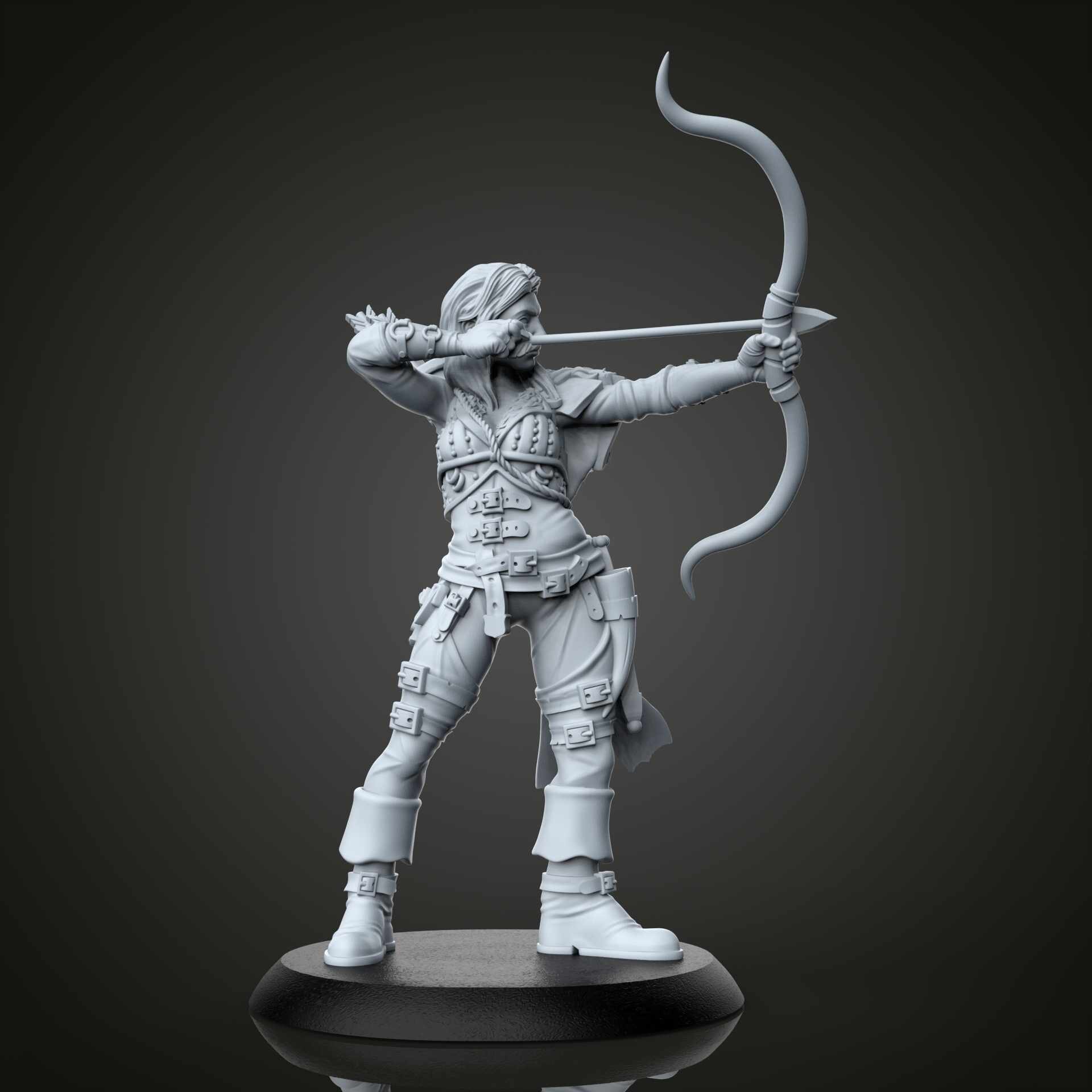This image showcases an intricately detailed sculpture of an archer, likely made from a hard plastic or porcelain material, with a light blue to off-white hue. The archer stands poised on a black, disc-shaped platform with another base beneath it. The background is a textured dark gray with subtle white patterns that resemble a delicate sunburst effect. The archer, whose gender appears indistinct due to slight variations in the captions, is depicted wearing a detailed uniform. This includes a vest, several belts around the waist and hips, white boots with large cuffs, and white pants. The archer's attire features additional accessories like epaulets on the shoulders and what appears to be a crest on the vest. The figure has long hair that extends down the back and a potential mustache, although this could be obscured by other details.

In a dynamic pose, the archer pulls back the string of a curved bow with the right hand, ready to release an arrow held just above the left hand, which grasps the bow's center. This meticulous piece of art captures both the tension of the archer's draw and the calm confidence in their stance, brought to life through the detailed craftsmanship and textured background.